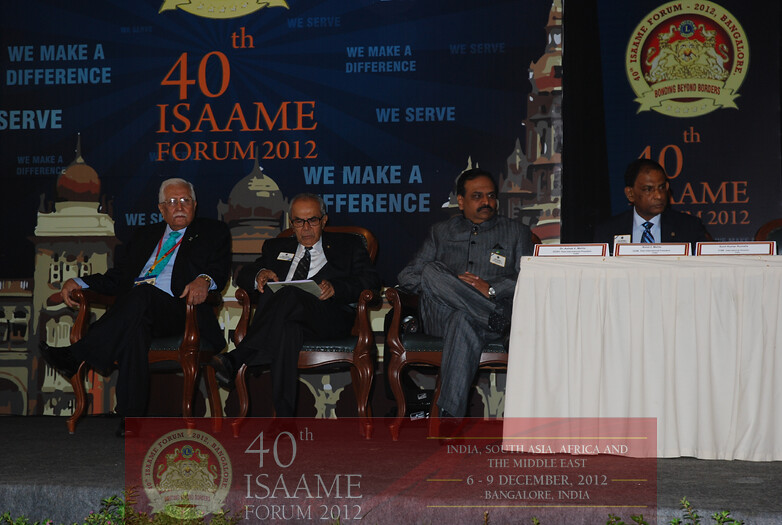The image shows four well-dressed men seated on a stage during the 40th ISAM Forum 2012 held in Bangalore, India from the 6th to the 9th of December. Three of the men are in polished, decorative wooden armchairs, dressed in black and gray suits with white dress shirts and ties. The fourth man sits behind a table draped with a white tablecloth, featuring a name tag. Behind them, a poster adorned with images of Indian temples or palaces reads "40th ISAM Forum 2012: We make a difference, we serve," in blue font, along with regions "India, South Asia, Africa, and the Middle East" and event details. An additional red overlay at the bottom echoes these details, emphasizing the forum's international focus and celebratory nature.